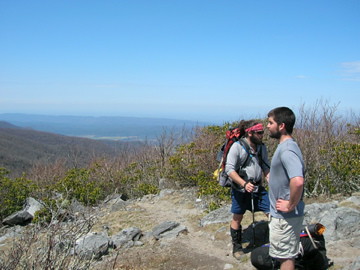The photograph captures two bearded men, likely in their mid to late 20s, standing on a rocky, dusty path atop a mountainous area with a sweeping view of the landscape. One man, positioned in the front, wears a gray short-sleeve t-shirt, beige shorts, and stands with his hands on his hips, gazing at the expansive scenery. His black boots are visible and his backpack rests on the ground nearby. The second man, slightly behind, sports a gray long-sleeve shirt, dark blue shorts, long black socks, and a red bandana, and he carries a backpack on his shoulders. Both men are surrounded by an assortment of stones, leafy and dry shrubs, and grasses. The distance reveals a sprawling low valley with additional hills and mountains stretching towards a clear, pale blue sky devoid of clouds.